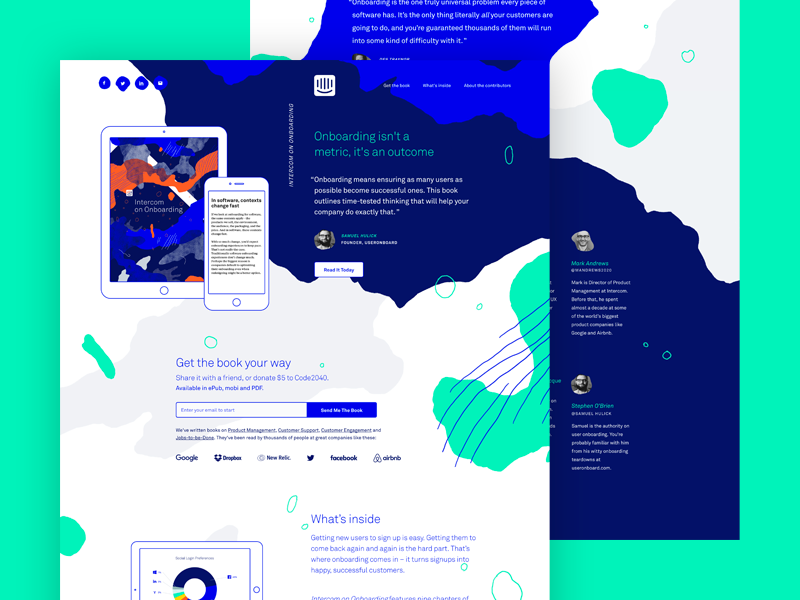The page displays a vibrant and informative design focused on the theme of onboarding. At the top, bold green text reads, "Onboarding isn't a metric, it's an outcome." Below, in white text, it states, "Onboarding means ensuring as many users as possible become successful ones. This book outlines time-tested thinking that will help your company do exactly that." This quote is attributed to the founder of the company, although the name is difficult to discern due to the small, low-resolution text.

Centrally, there is a prominent white button labeled "Read it today." To the left, the interface examples show how the content appears on both an iPad and a phone. Below this, a section encourages readers to "Get the book your way, share it with a friend, or donate $5 to Code2020." This call-to-action is accompanied by an open input field and a blue button that says "Send me the book."

Additionally, logos of prominent companies such as Google, Dropbox, New Relic, Twitter, Facebook, and Airbnb are displayed, lending credibility and indicating industry relevance. Another highlighted section asserts, "What's inside: getting new users to sign up is easy, getting them to come back again and again is the hard part. That's where onboarding comes in; it turns signups into happy successful customers."

The overall design features a white background with strategic splashes of blue and green, creating an engaging visual experience. The entire image is bordered by a complementary green, adding to the cohesive aesthetic.